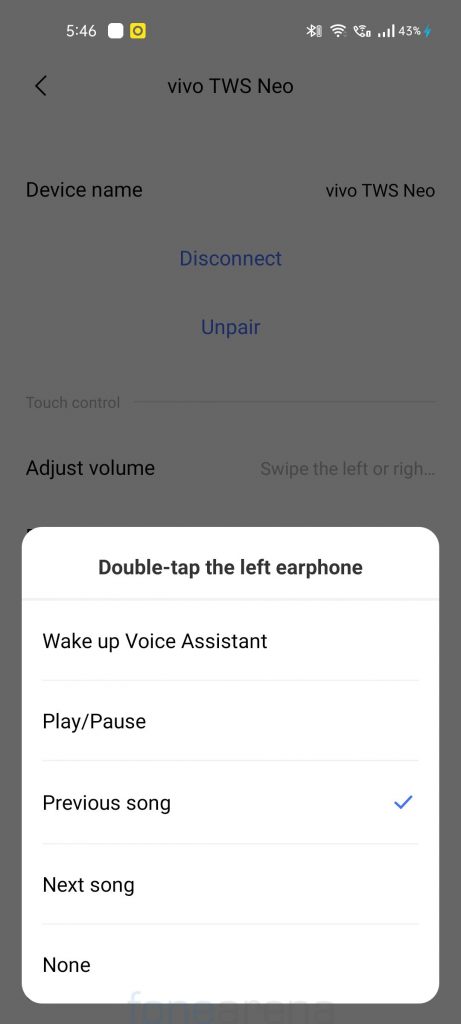This image appears to be a screenshot of a smartphone displaying a settings page for a Bluetooth device. The background is predominantly gray. At the very top, the status bar shows the time as 5:46 in white text. To the right, icons display signal strength with five bars, a 43% battery life, and Wi-Fi connectivity, all in white.

Beneath the status bar, the name "Vivo" is displayed in black uppercase letters, and next to it "TWS neo" in a mix of upper and lower case. Preceding this text is a left-pointing arrow (less than sign without a horizontal line behind it). Below this, the words "Device Name" are also in black, and further to the right, "Vivo TWS neo" is repeated. Between these two sets of words, there is a considerable amount of space occupied by the options "Disconnect" in blue text and "Unpair" following a small gap.

Moving down, on the far left, the text "Adjust volume" appears in black. To the right of this, in a slightly darker gray than the background, it instructs to "Swipe left or right," followed by a series of ellipses indicating continuation.

Below, a white and red-bordered square with smoothed corners at the bottom contains further instructions. At the top, "Double tap" appears in small black font, clarifying that the message relates to the left earphone. Below this, in black font, the actions listed are: "Wake up voice assistant," "Play/Pause," "Previous song" with a small blue check mark to the right indicating selection, "Next song," and "None."